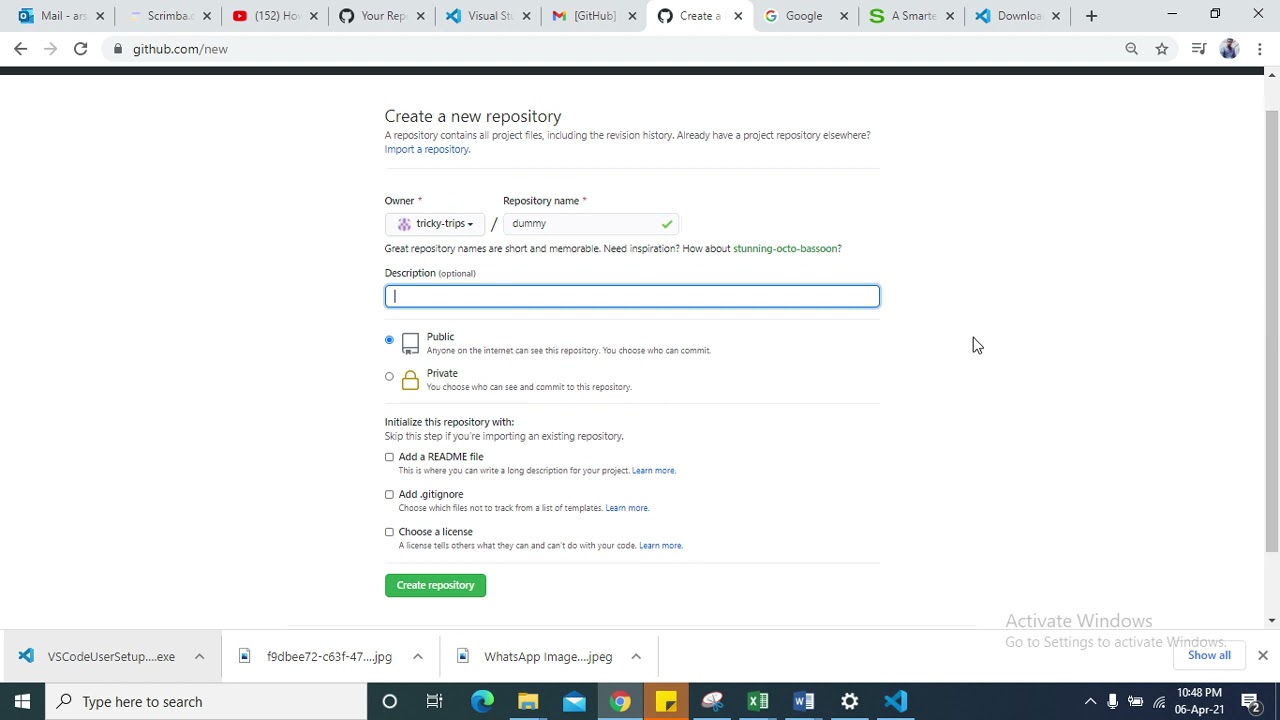A screenshot showcases a computer screen, potentially from a laptop or a workstation, with around 10 tabs open across the top. The active tab displays a URL in the address bar: github.com/new. The visible web page is titled "Create a New Repository," and provides general information about what a repository is. Below this are several interactive options for setting up the new repository: fields for entering a description, toggles for making the repository public or private, and additional customizable options such as adding notes and themes. Although one of the options is not clearly readable, the form ultimately culminates in a prominent green button labeled "Create Repository" at the bottom.